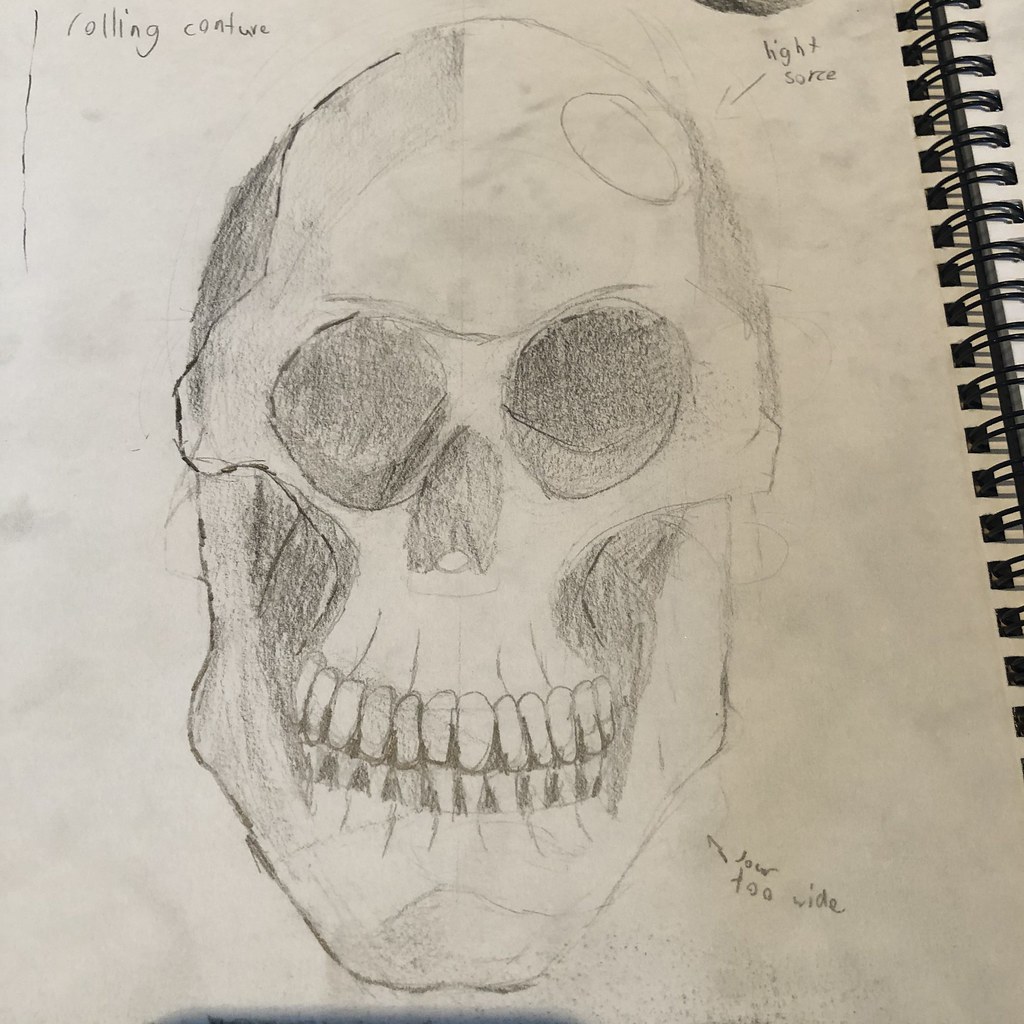This is a detailed drawing of a human skull done on white paper in a spiral-bound sketchbook, likely by a student with more skill in drawing than in writing. The drawing is annotated with various labels, suggesting an educational context. The skull, which is wider than a typical human skull and asymmetrical, features detailed work including all its teeth—both top and bottom, and more than a normal human would have. There is a notable shading effect on different parts of the skull: the eyes, cheeks, nose, and some of the back are shaded, indicating depth and light source. 

Around the skull are several annotations in a child's handwriting, including one at the top left corner of the page that reads "rolling contour," although the first letter might be unclear. Another label on the upper right points to the right side of the skull, saying "light source," which correlates with the lighter shading on that side. At the bottom right, an arrow points to the jaw and is labeled "jaw too wide," criticizing the discrepancy between the size of the jaw and the upper part of the skull. Additionally, on the top of the skull, there is a large circle that appears to depict a hole. The overall impression is that of a student's draft for an art class, with various notes indicating areas for improvement.